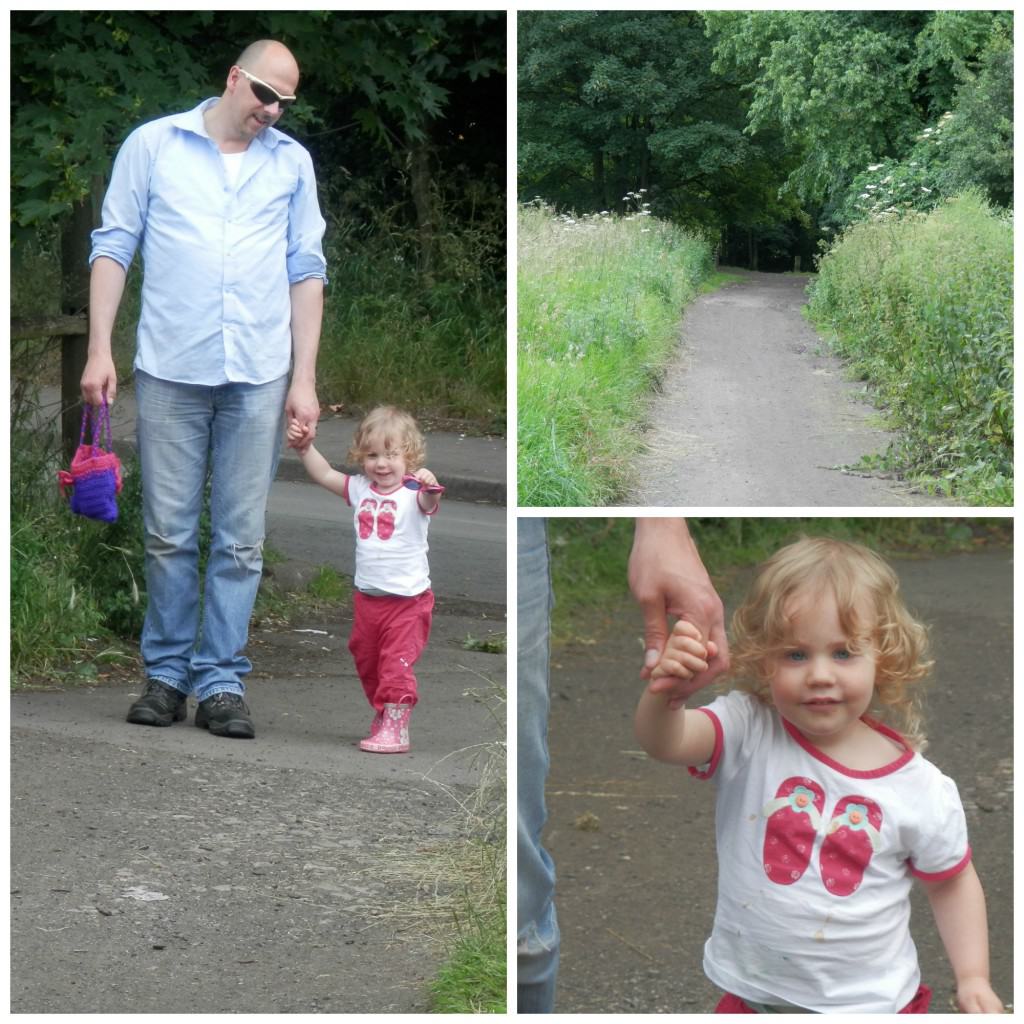This is a composite of three color photographs: a large vertical image on the left side and two smaller square images stacked vertically on the right. In the main image on the left, a man and a young girl are depicted holding hands while looking at the camera. The man, wearing a light blue, button-down shirt with rolled-up sleeves, blue jeans with holes at the knees, and black sneakers, is also holding a purple and dark pink knitted or crocheted bag in his right hand. His left hand is clutching the hand of the child. He’s balding, wearing Oakley sunglasses, and looking down at the girl. The little girl, with blonde curly hair and blue eyes, is wearing a white short-sleeve shirt adorned with pink ovals or perhaps tiny illustrations and trimmed in pink around the collar and sleeves. Her pink windbreaker pants and pink rain boots complete the outfit, and she’s holding a pair of pink sunglasses in her left hand. They are standing on a gray asphalt road bordered by lush green brush and trees on either side.

The top right photograph is of the same road seen in the left image, devoid of people, highlighting the path as it stretches forward, flanked by dense greenery. The bottom right photograph zooms in on the girl, capturing a close-up of her looking at the camera. Only the father's leg and hand are partially visible, holding the girl's hand. The concrete walkway, present in the main image, serves as the background.